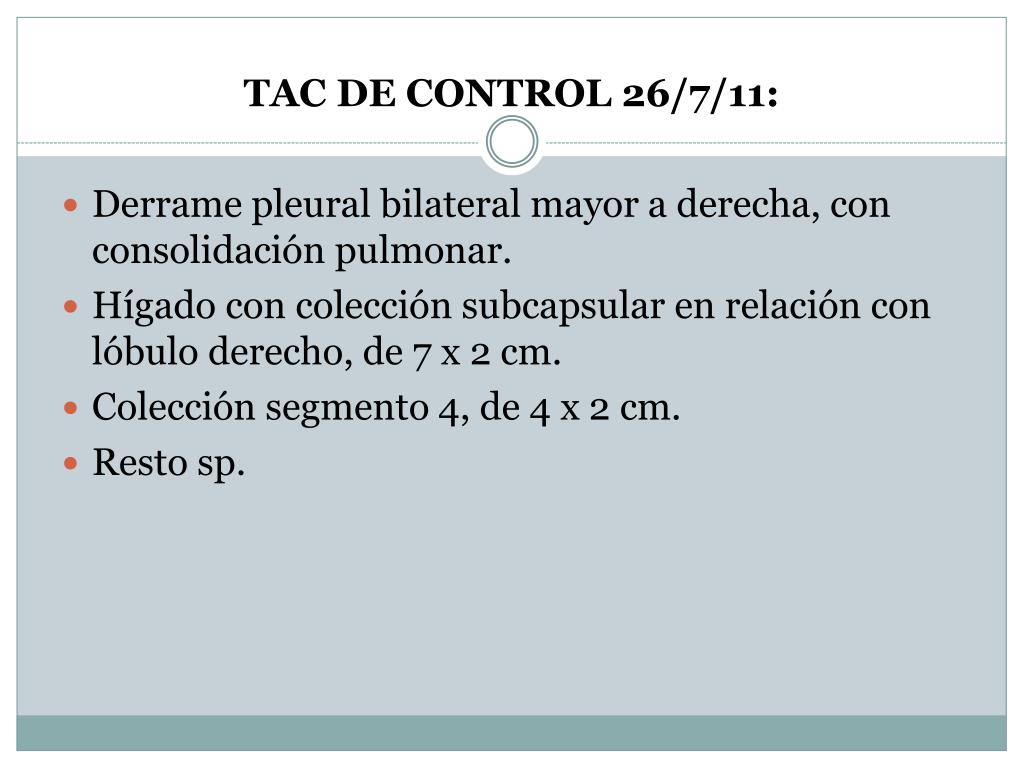This image of an informational page features a PowerPoint slide. The top section has a white background outlined in light blue with black text in all caps reading "TAC-DAY CONTROL 26/7/11:". Below this, a large rectangular area has a solid gray background with four red bullet points, all left aligned and in black text. The bullet points are:

1. "DERAME PLURAL BILATERAL MAYOR A DERECHA CON CONSOLIDACION PULMONAR"
2. "HIGADO CON COLECCION SUBCAPSULAR EN RELACION CON LOBULO DERECHO DAY 7-X-2-CM"
3. "COLECCION SEGMENTO 4, DAY 4-X-2-CM"
4. "RESTO SP."

The entire text appears to be in Spanish. At the very bottom of the image is a narrow, horizontal, darker gray section. Additionally, there is a unique element at the top: a white circle enclosed by two larger teal circles situated just below the word "CONTROL".